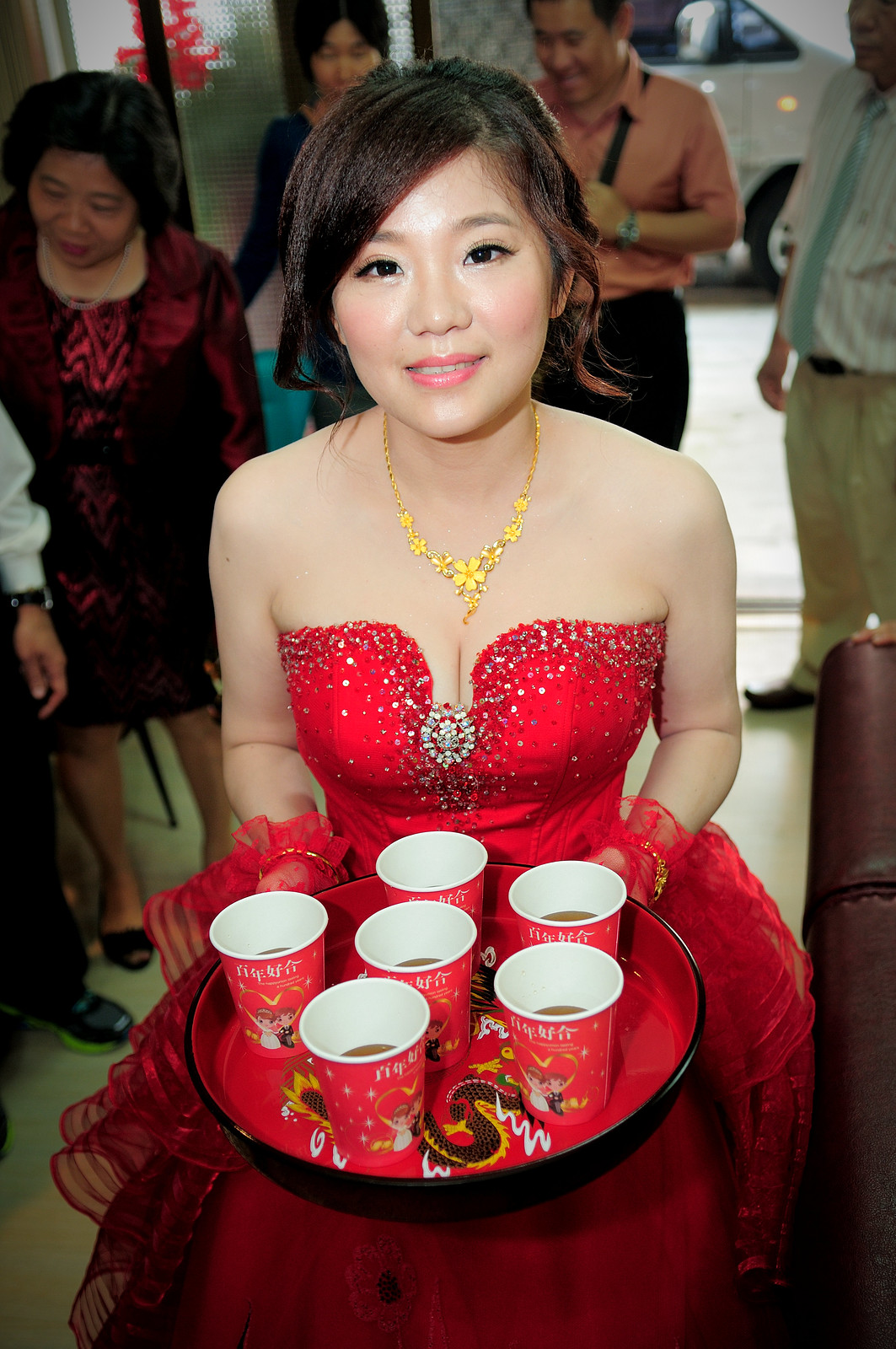This photograph captures an elegant Asian woman, adorned in an exquisite strapless red gown intricately embellished with rhinestones. The gown features a bustier and is accentuated with a silver pendant and jewelry at the center, as well as red lace gloves on her hands. The long, layered skirt has netting and taffeta, with ruffles around her wrists but does not extend to the floor. Her hair is styled in an updo, potentially in a bun, and she wears eye makeup, light pink lipstick, and a gold necklace with a floral centerpiece.

In her hands, she holds a circular black tray lined with red paper, featuring a prominent dragon design. The tray carries six reddish paper cups, adorned with illustrations of two children and possibly dragons, each partially filled with a brown liquid—perhaps coffee or cola. This scene takes place at a vibrant event, evidenced by the background where more Asian individuals are present. Many of them appear to be engaged with their phones, and not focused on the camera, while a few are smiling. The color palette in the image includes reds, blacks, beiges, and flesh tones, with some attendees wearing distinctive outfits such as a gentleman in a teal tie with a white-striped shirt and light green pants, and another in an orange short-sleeved collared shirt paired with black pants.